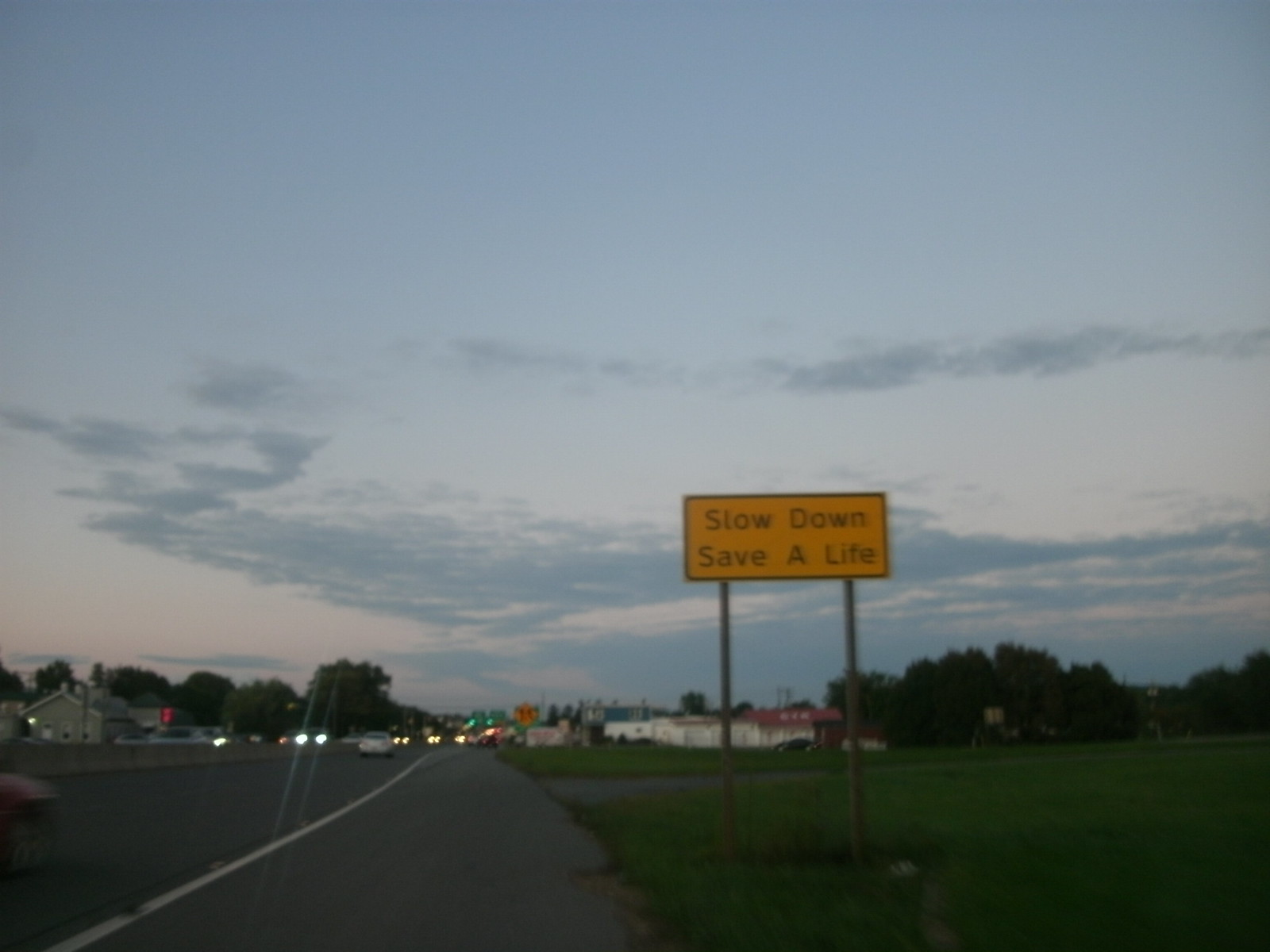This is an image taken from the shoulder of a road at dusk, where a faint blue sky with some clouds is still visible, but the sun has set. The road is divided into two lanes by a white line, with a few cars in the distance, their headlights illuminating the darkening scene. To the left of the road, a concrete barricade separates the oncoming traffic, including a visible white car with its headlights on. On the right side of the road, there is a grassy patch with a rectangular yellow sign that reads "Slow Down, Save a Life," held up by two poles. This sign is in the foreground, approximately 15 feet from the observer, who seems to be standing close to it. Further down the road, on the right, are some distant buildings, including a white one, and scattered trees. An orange diamond sign indicates a merging lane ahead, and in the far distance, a traffic light glows green. There is also a little beige house to the left, adding to the suburban landscape. The scene captures the transition from daylight to night, as vehicles navigate the road under the gradually dimming sky.